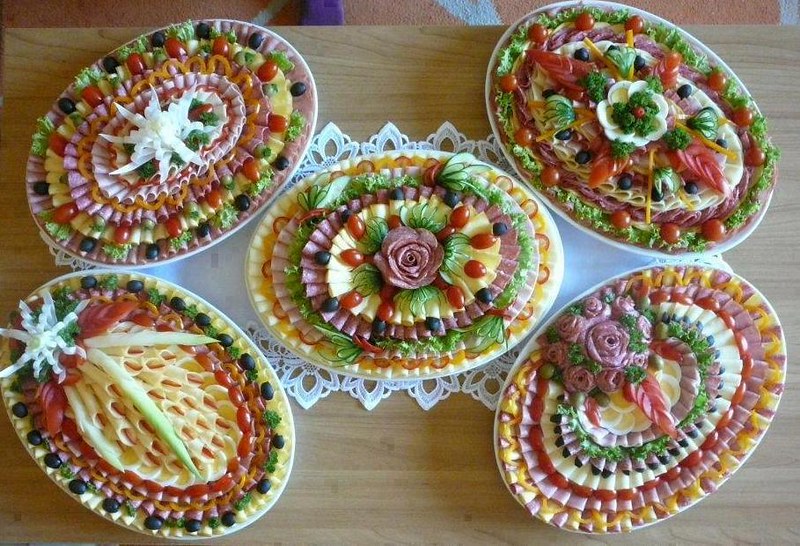This top-down photograph captures an intricate arrangement of five elaborate party platters artistically displayed on a light brown wooden table. Each large, oval-shaped bowl is meticulously crafted with layers of rolled cheese and various meats, forming distinct decorative patterns. The centerpiece platter is horizontal, flanked symmetrically by two platters on each side, angled to create a cohesive visual design.

Each platter showcases its own unique theme with different artistic designs. Highlights include rolled cheese resembling a pineapple, meats folded into rose shapes, and layered assortments featuring a variety of colors and textures. Some platters have decorative layers of egg yolks, lettuce, blueberries, and cherry tomatoes, adding vibrant reds, greens, whites, yellows, and pinks to the presentation. The outer edges are adorned with different meats, cheeses, and garnishes, forming elaborate spirals and floral patterns.

Beneath this culinary artwork, a white lace doily with a rectangular, lace-bordered design subtly peeks out, primarily under the central platter and partially under the side platters. On the beige and brown-toned table, additional elements like olives, tomatoes, and cucumbers are intricately placed to heighten the decorative appeal. Hints of purple are visible beneath the table, adding a mysterious touch to the vivid, colorful display.